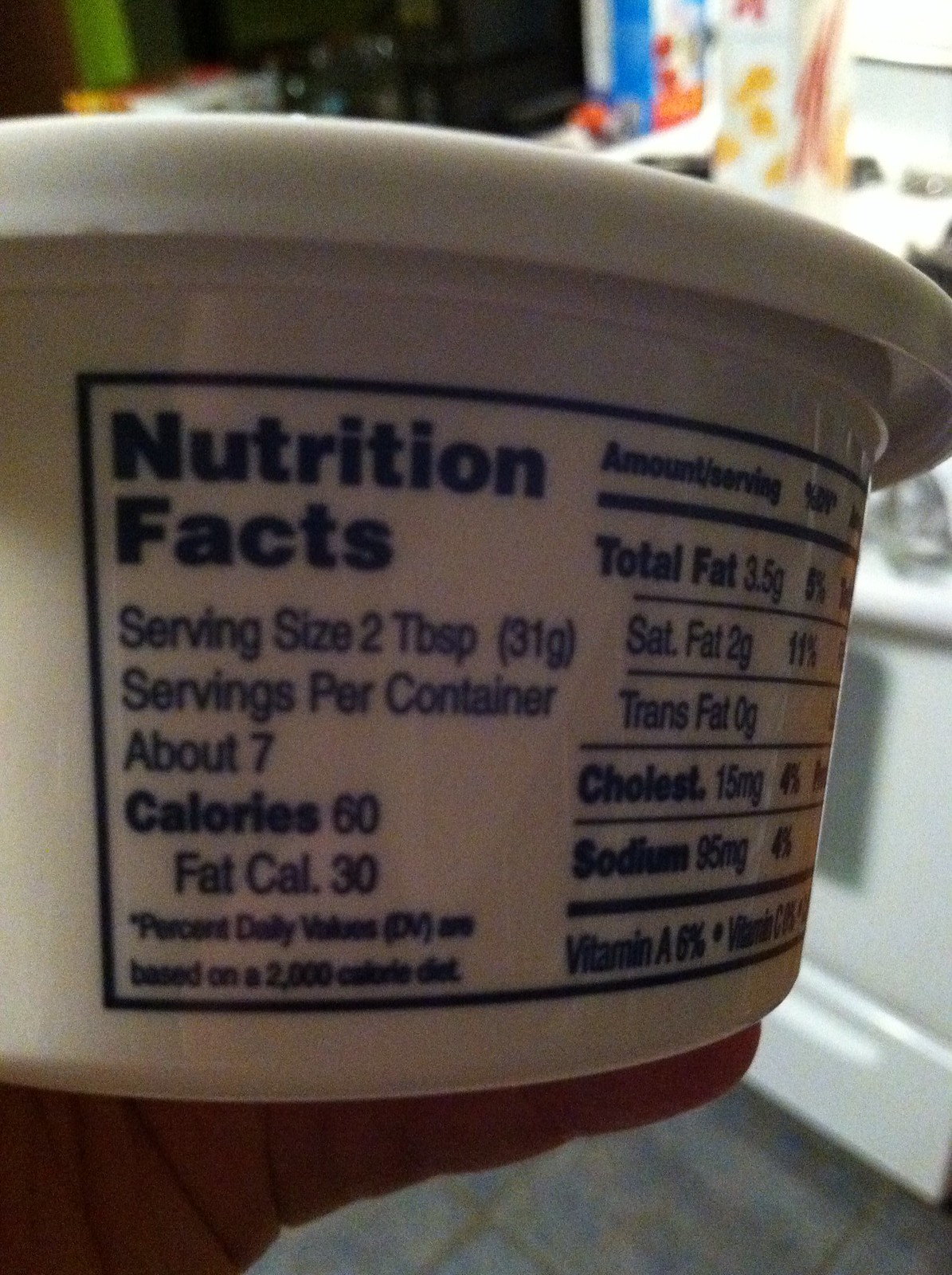This image is a close-up photograph of a white plastic round container with a prominently displayed Nutrition Facts label in blue ink. A person's finger is holding the container, which occupies most of the photo. The container has a lid and is positioned on a dark-colored counter. In the background, a portion of a white stove with a gray door and part of a tile kitchen floor are visible. Additionally, there seem to be multicolored curtains on a window. 

The Nutrition Facts label details the following: serving size is 2 tablespoons (31 grams), with about 7 servings per container. Each serving has 60 calories, with 30 coming from fat. Underneath, it lists various nutritional components: total fat is 3.5 grams, saturated fat is 2 grams, trans fat is 0 grams, cholesterol is 15 milligrams, sodium is 0.25 milligrams, vitamin A is 6%, and vitamin C, although the amount is unreadable. The Percent Daily Values are based on a 2,000-calorie diet. The specific product inside the container is not indicated.